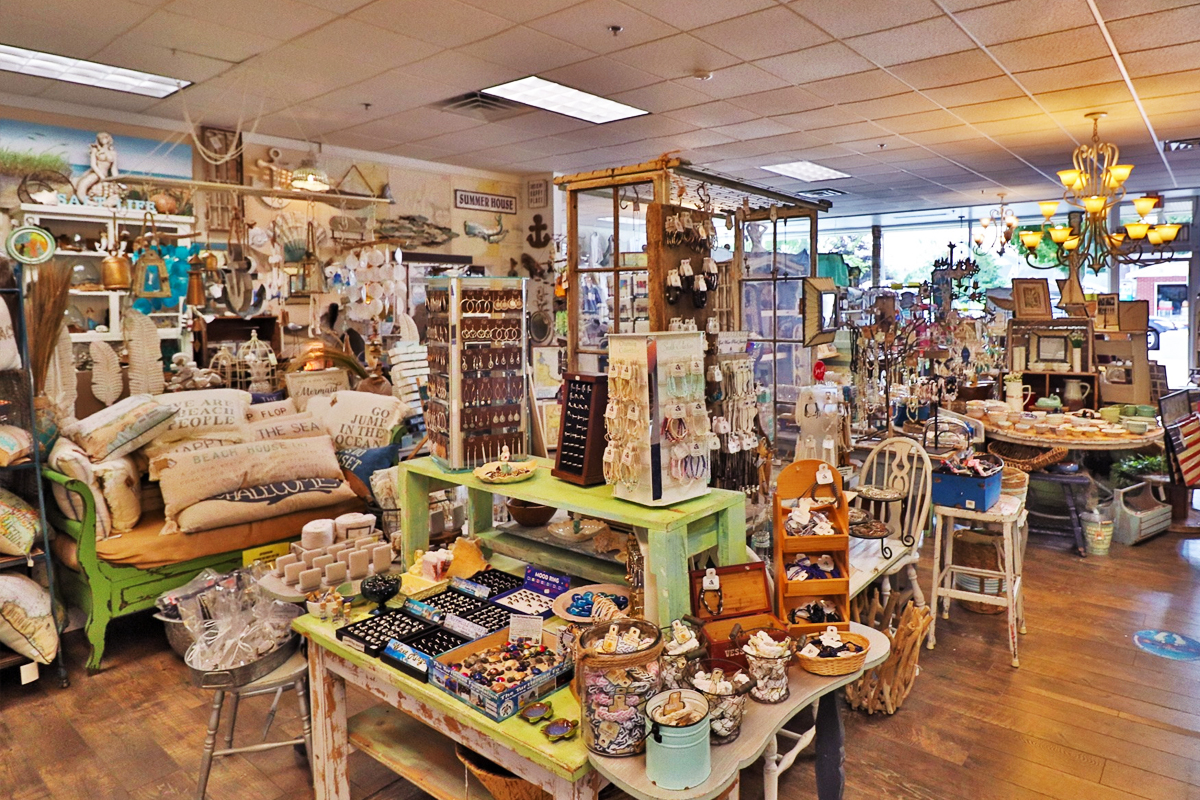The image depicts the interior of a charming and eclectic retail store, filled with an extensive variety of items that blend the whimsical feel of a tchotchke shop with the allure of a collector’s haven. The point of view is from the front of the store, offering a panoramic view of the space. In the foreground, a weathered white wooden table with a lime green riser is adorned with an array of jewelry, including earrings, rings, and bracelets. To the left, an ornate couch is piled high with a diverse assortment of decorative pillows. The right side of the shop features a round table brimming with teacups, bowls, and other decorative items, while in the background, another table showcases additional jewelry pieces. The space is lit by a grand chandelier hanging from the white ceiling. Rustic and vintage decor elements, such as wooden boxes, glass bins filled with thread and candles, and shelves made from old barn windows, add to the store’s quaint charm. Multiple tables are set up with various collections of antiquities, wall art, and decorative furniture, suggesting that the shop may offer rented sections for different crafters or collectors to display their wares. The front of the store is lined with large windows, allowing natural light to illuminate the diverse and colorful merchandise within this captivating and bustling space.